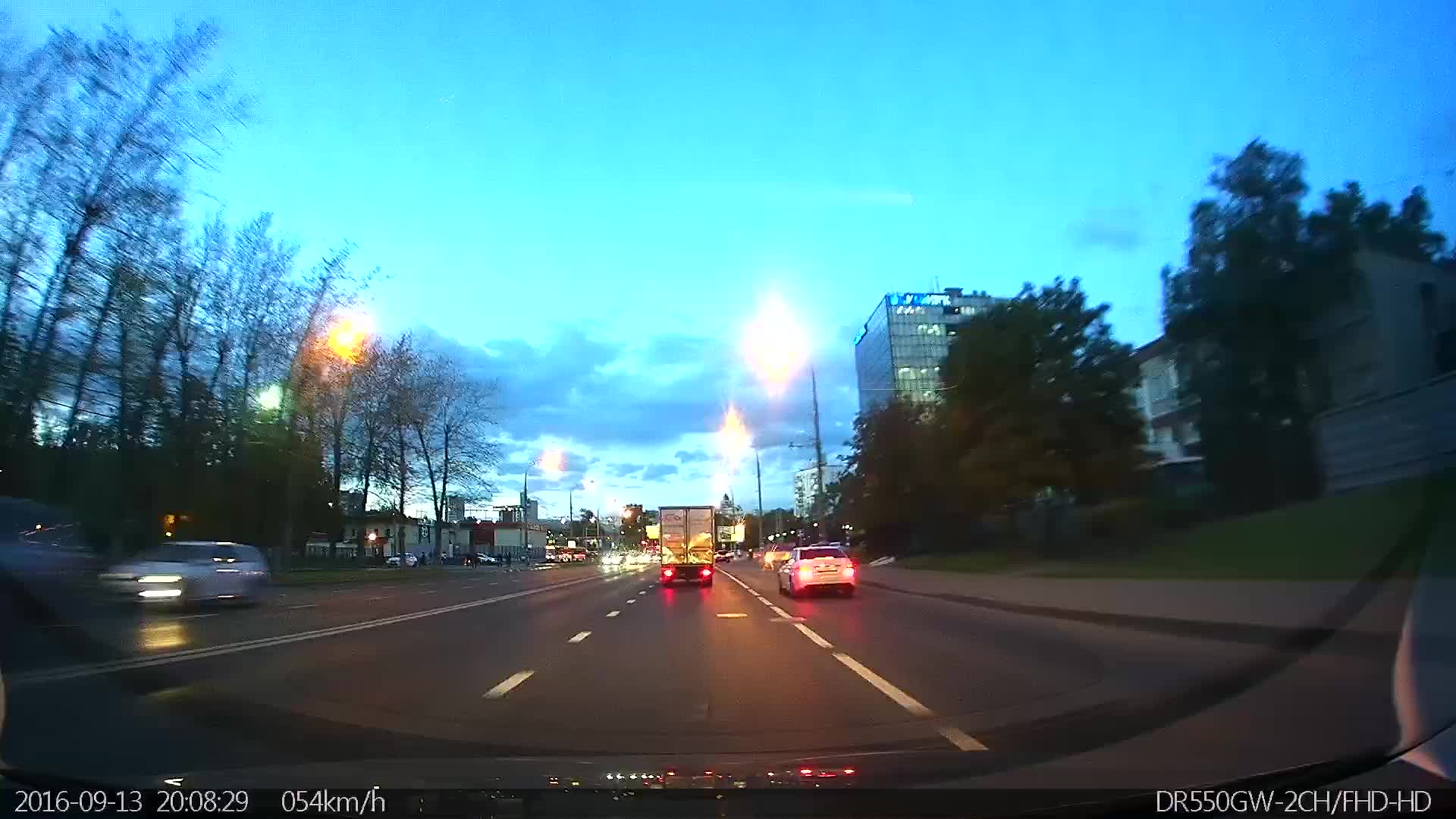The image, captured on September 13th, 2016, at 8:08:29 p.m., depicts a scene from the perspective of a car traveling at 54 kilometers per hour along a three-lane road in an urban environment. The image, taken from a dash cam, shows a typical fish-eye lens view with date, time, and speed information displayed at the bottom. The roadway is busy, with three lanes of traffic moving in each direction.

It is dusk, as indicated by the dim blue sky and the presence of fully illuminated street lamps. Cars, including a semi-truck directly ahead in the middle lane and a white car in the right lane, have their headlights on, reflecting the low-light conditions. The photograph captures buildings in the background, including a cubic, blocky apartment building to the right, with some shops further down the street. The streetscape is bordered by sidewalks, short green grass, and rows of trees, creating a blend of urban and natural elements.

Overall, the scene portrays a typical city road at dusk, characterized by moderate traffic, illuminated street lamps, and a mix of residential and commercial buildings set against a backdrop of twilight and deepening clouds.